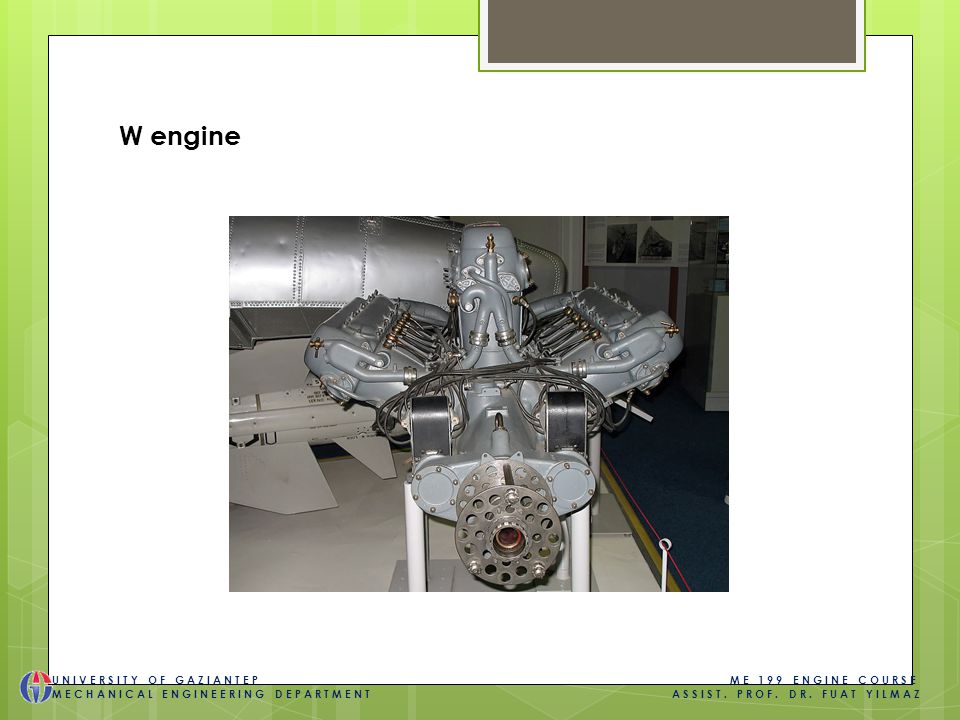The image is a detailed photograph of a large, intricate engine, predominantly silver or gray in color with gold-colored components. The engine appears to be on display, possibly in a museum or exhibit room, suggested by the surrounding items like airplane parts visible in the background. The engine is placed on a partially white-tiled floor, with adjacent darker gray tiles on the right side. The background features shelves and boxes.

The image itself is framed with a bright green border surrounding a solid white background. At the top left of the white background, the designation "W Engine" is written in black text. The bottom left corner of the image includes a printed label stating, "University of Gaziantep Mechanical Engineering Department," and the bottom right corner reads, "ME 199 Engine Course Assist Professor Dr. Fuat Yilmaz." This suggests the engine is used for academic purposes within the University's Mechanical Engineering Department and likely features in a course taught by Assist. Prof. Dr. Fuat Yilmaz.